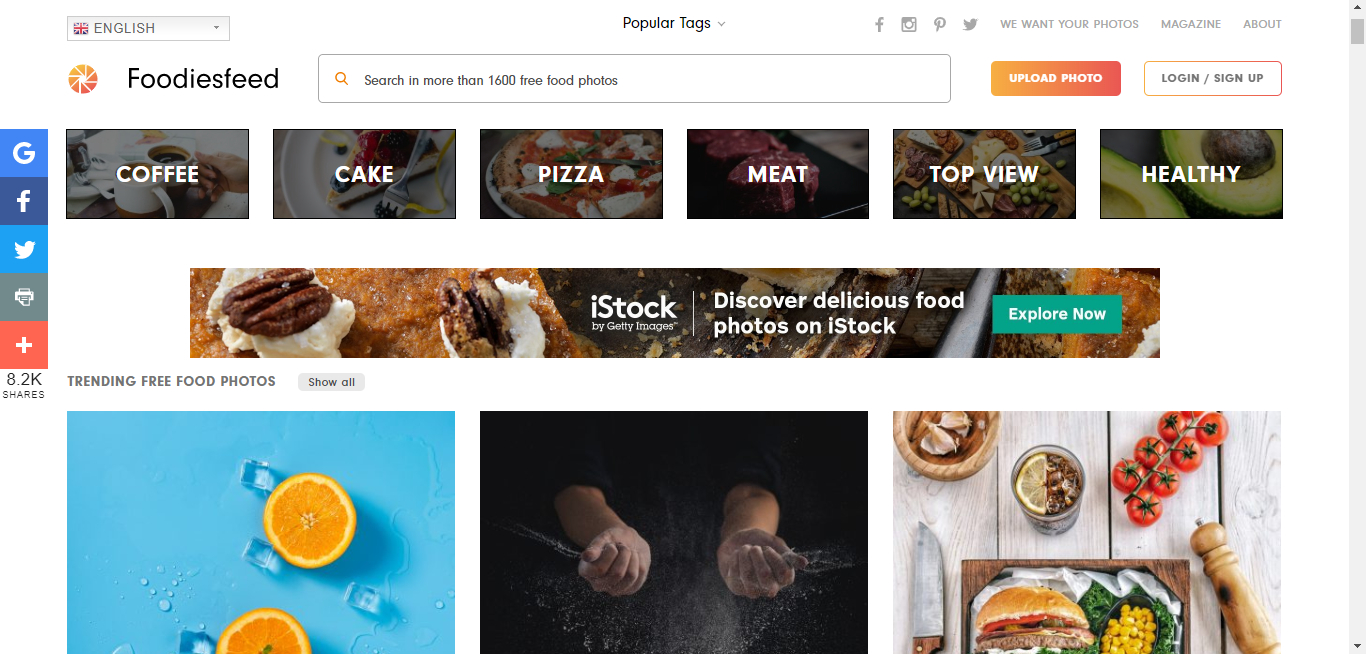This is an image of the Foodies Feed website, designed with a pristine white background. Dominating the right side of the page is a vertical, elongated scroll bar, enabling intuitive navigation both via mouse drag and clickable functionality.

Starting from the top left corner, the website offers a language selection option. Centrally positioned, "Popular Tags" is prominently displayed, flanked by social media icons for Facebook, Instagram, Pinterest, and Twitter. Adjacent to these are three key links: "We Want Your Photos," "Magazine," and "About."

To the left, the brand name "Foodies Feed" is elegantly presented, accompanied by a compact company logo to its right. A central feature is the expansive search bar, inviting users to "Search in more than 1600 free food photos." Beside this, two buttons are visible: "Upload Photo," distinguished by its orange and peach background, and "Login and Sign Up," with a contrasting white background.

Below, a selection of buttons, each paired with a representative background image, is displayed. These include categories such as:
- **Coffee:** Illustrated by a hand holding a coffee cup.
- **Cake:** Depicted with a cheesecake image.
- **Pizza:** Displayed with a delectable pizza.
- **Meat:** Shown with an image of succulent meat.
- **Top View:** Accompanied by top-view food photography.
- **Healthy:** Featuring an image of avocados.

To the left of this segment, a smaller vertical bar hosts social media share icons for Google, Facebook, Twitter, and possibly print or email, culminating in a plus sign. This section indicates a total of "8.2k shares."

Further below, a horizontal bar showcases an enticing food photo backdrop overlaid with the text "iStock by Getty Images." The accompanying caption reads, "Discover delicious food photos on iStock," followed by an "Explore Now" button to the right.

The bottom segment displays three partially visible images:
1. **Orange slices:** Arranged with small ice cubes on a blue surface.
2. **Flour sprinkle:** Capturing a hand sprinkling flour against a black backdrop.
3. **Assorted food items:** Featuring a pepper grinder, a burger with salad, iced tea, tomatoes, and a knife on a wooden table.

This thorough layout and design evoke a sense of culinary exploration, inviting users to delve into a variety of visually captivating food photographs.